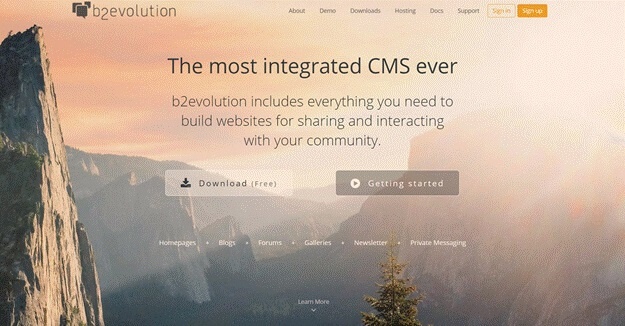A stunning mountain landscape bathed in light is the centerpiece of this image. The sky exhibits a gradient from a peachy orange hue on the left to a brighter, lighter tone on the right, creating a serene atmosphere. The silhouettes of the mountains appear in a gray-blue shade, adding depth and contrast to the scene. 

In the upper left corner, three overlapping speech bubbles with gray backgrounds and white outlines display the characters "b," "2," and "evolution" sequentially. To the right of these speech bubbles, a series of navigation buttons are neatly lined up, labeled: About, Demo, Downloads, Hosting, Docs, Support. Further right, two prominent buttons catch the eye: an orange-outlined rectangle with the label "Sign In" in orange text, and a solid orange rectangle with "Sign Up" in white text.

Dominating the center of the image, bold lettering announces: "The most integrated CMS ever." Below this, a smaller text elaborates, "B2Evolution includes everything you need to build websites for sharing and interacting with your community." Towards the bottom, there are two call-to-action buttons. To the left, a white rectangle featuring a download symbol and the word "Download" with "Free" in parentheses. To the right, a gray rectangle with a circular icon and a right-pointing arrow, labeled "Getting Started."